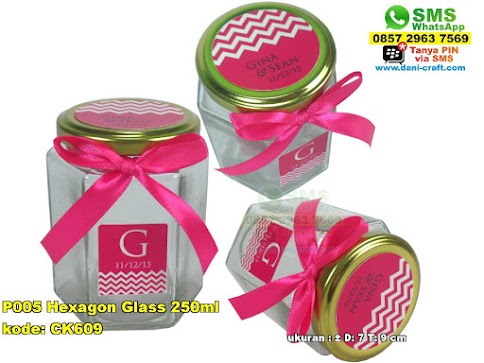The image is a product advertisement featuring three hexagonal glass jars, each adorned with a pink ribbon bow around the neck. The jars are arranged in various positions: the jar on the left stands upright, the one at the top is tilted to the left showing its gold lid, and the one in the bottom right corner lies on its side. Each jar has a gold lid with a circular pink label featuring white zigzag lines and the text "Gina and Sean" along with the date "11/12/15." The clear glass of the jars reveals a thick, sturdy structure, with a pink label on the front carrying a large white "G." The background is completely white, giving the impression that the jars are floating. Additional text appears in the bottom left corner of the image, detailing product specifications: "P005 hexagon glass, 250 milliliter code K9609" in yellow, along with contact information in various colors and fonts including a green SMS WhatsApp number, a red star, and a website URL, "www.dannycraft.com".